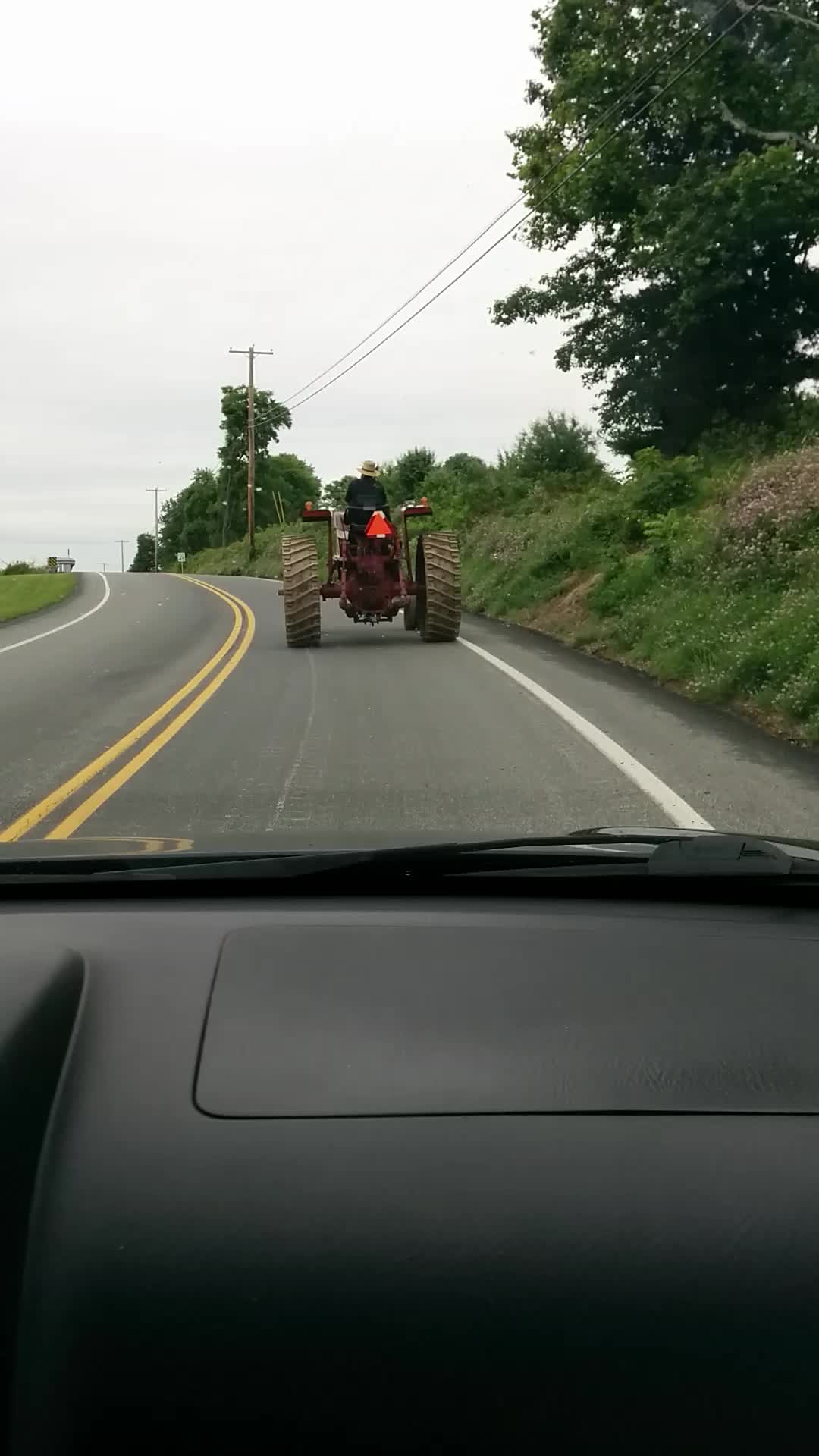A tall, rectangular photograph captures a scene from the passenger side of a vehicle, looking ahead through the windshield. Prominently in view is the back of a large tractor driving down a two-lane road, just a few car lengths ahead of the vehicle. The tractor features sizable, dirt-covered tires and an orange triangular warning sign affixed to its rear. The bottom of the image shows a portion of the vehicle's black dashboard. To the right, a steep, grassy embankment rises, dotted with tall grass and bushes. At the top of this embankment stands a solitary large tree, with power lines stretching along the road in the distance. The overcast sky adds a sense of dreariness to the scene.